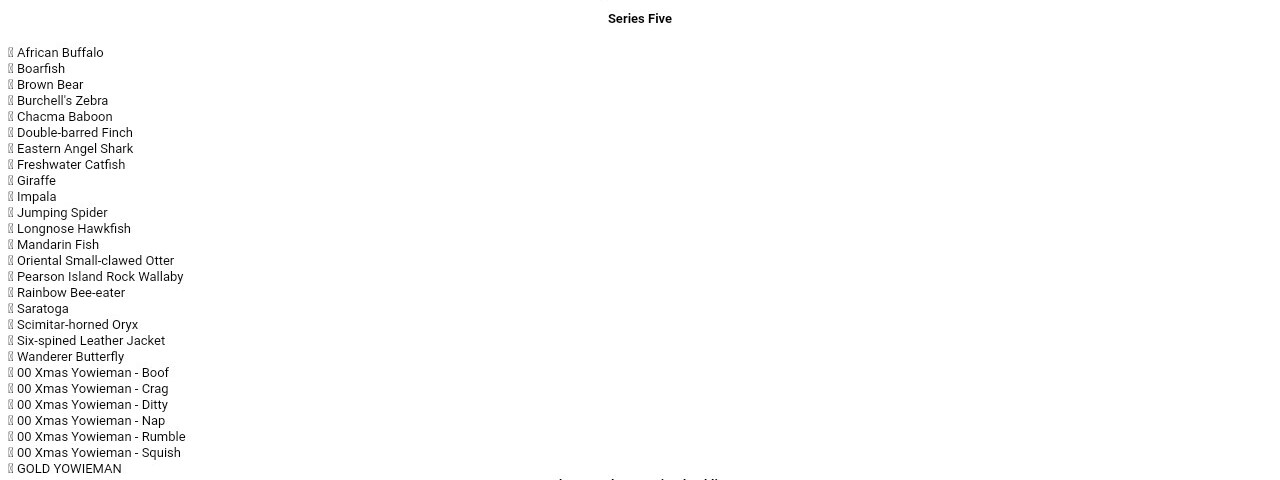A wide, minimalist page titled "Series 5" appears on the right side against a stark white background. On the left side of the image, a long and detailed list of various animals is presented in small, hard-to-read black text. The extensive list features creatures like the African buffalo, boarfish, brown bear, virtual zebra, baboon, finch, shark, freshwater catfish, giraffe, impala, and jumping spider. Towards the bottom, more peculiar names such as the six-spined leather jacket and various forms of "yowieman" (e.g., x-mas yowieman) are included. Despite the detailed inventory of animals, the image lacks contextual information and is dominated by an excessive amount of blank space, lending to a rather plain and ambiguous appearance.